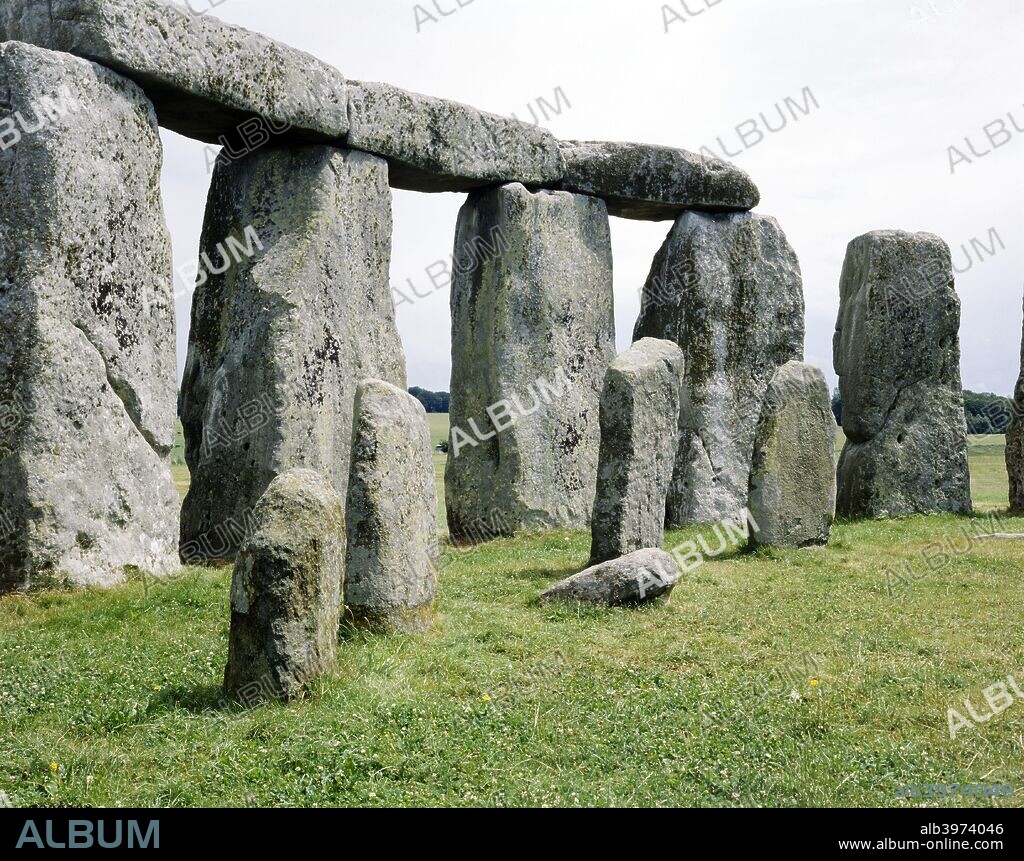The image captures the iconic Stonehenge formation set in a grassy clearing during a partly cloudy day. Five massive stone pillars stand upright, arranged in a circular pattern, with large horizontal stones resting atop the first four, forming a series of ancient dolmens. In the foreground, five smaller stones are scattered, with the middle one leaning forward on its face. The backdrop features a softly overcast sky and a distant wooded area, providing a serene contrast to the stark, monumental stones. A black strip runs along the bottom of the image, displaying the word "album" on the left side and the text "ALB3974046" followed by the website "www.album-online.com" on the right. Additionally, the photograph is watermarked diagonally with the word "album" in both solid white and black letters on white.